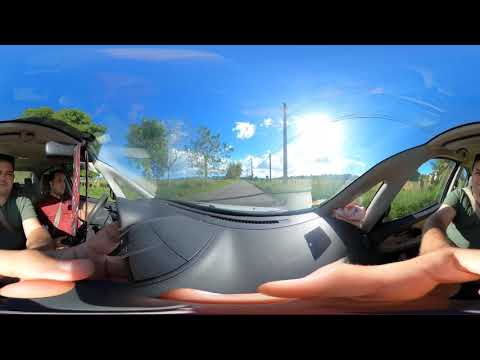This image captures two people sitting in a car, with the coupled distortion from the lens creating an unusually stretched and undulating appearance to the body parts, particularly the hands and fingers, as well as the car's interior. The scene is flooded with light from an overexposed sun flare that sits behind the blue sky dotted with clouds, visible through the windshield. Trees and power lines can be seen through the windshield, adding to the outdoor, sunny midday setting.

The image composition places the two individuals—the passenger's right half on the right side and their left half to the left—nestled into the bottom left corner. The person on the left appears to be a woman wearing a red shirt, while the older male passenger on the right is clad in a dark green shirt. Adorning the interior is a red and white ornament hanging beneath the rearview mirror, possibly an American flag.

The overall color palette includes black, blue, gray, white, green, red, tan, and silver tones. The solid black border frames the top and bottom of the image, encapsulating a scene of distorted human forms and an interior car space juxtaposed with a bright and cloud-filled sky.